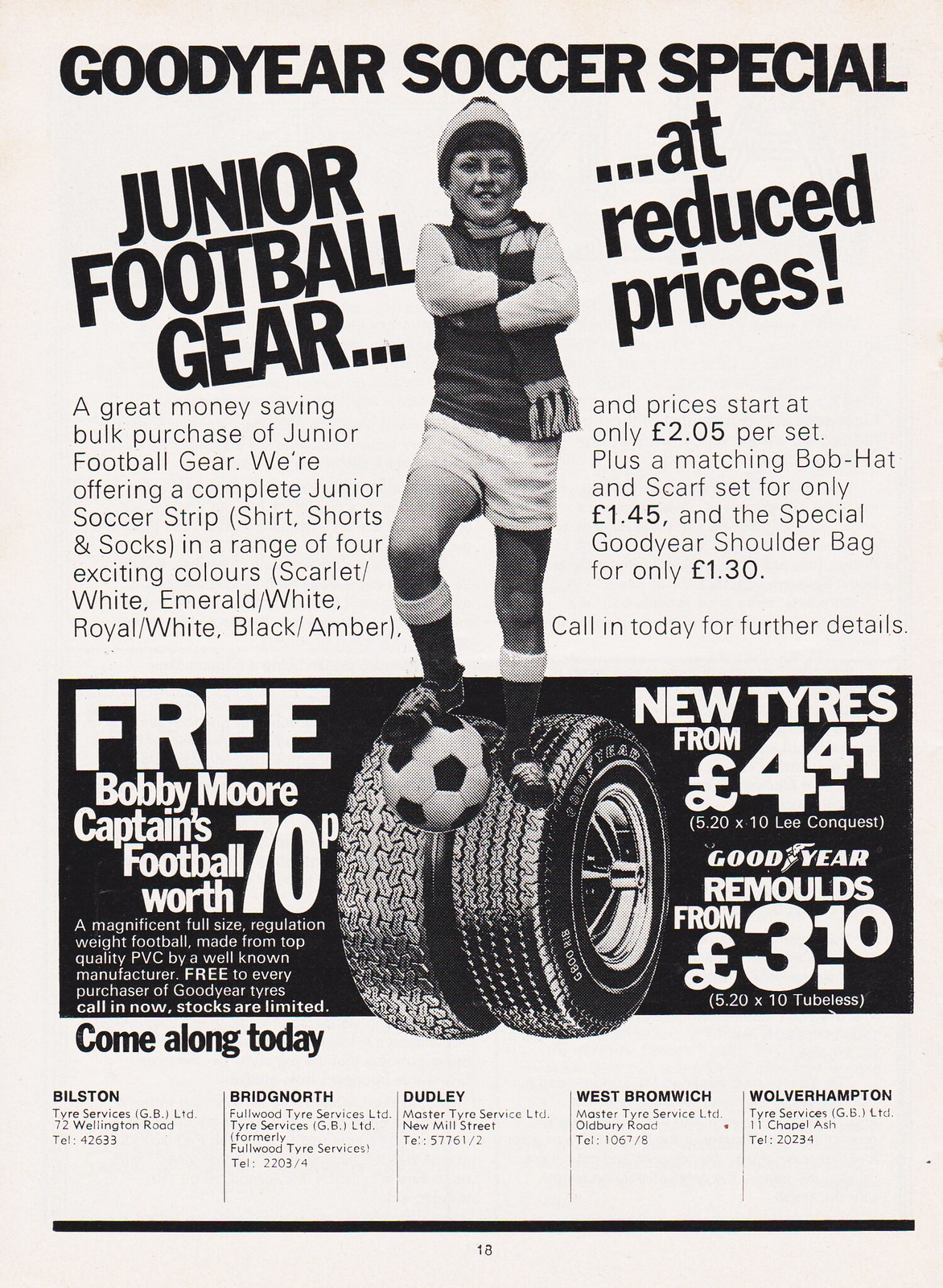This black and white scanned flyer advertises Goodyear's soccer special, highlighting junior football gear at reduced prices and offering a unique promotional blend with their tire products. At the very top, the flyer boldly states "Goodyear Soccer Special - Junior Football Gear at Reduced Prices," emphasizing a money-saving bulk purchase deal.

Central to the design is a digitally-inserted cartoon-like child, who is standing confidently with arms folded. The child, wearing a complete soccer strip that includes a jersey, scarf, and beanie, along with white shorts, has one foot placed on a soccer ball - an image that overlaps with a pair of prominently displayed large tires. The flyer mentions that the soccer gear comes in four vibrant color combinations: scarlet white, emerald white, royal white, and black amber.

Detailed pricing information is provided: sets start as low as 2.50 euros, with additional offers including a matching bob hat and scarf set for 1.45 euros, and a special Goodyear shoulder bag for 1.30 euros. There is also a special mention of a "free Bobby Moore captain's football" priced at 70p.

The lower portion of the flyer lists the locations of Bilston Bridge North, Dudley, West Bromwich, and Wolverhampton, and it includes a couple of paragraphs detailing pricing and a call-to-action for further details.

Finally, vibrant Goodyear logos are displayed, offering new tires starting from 4.41 euros and remoulds from 3.10 euros.